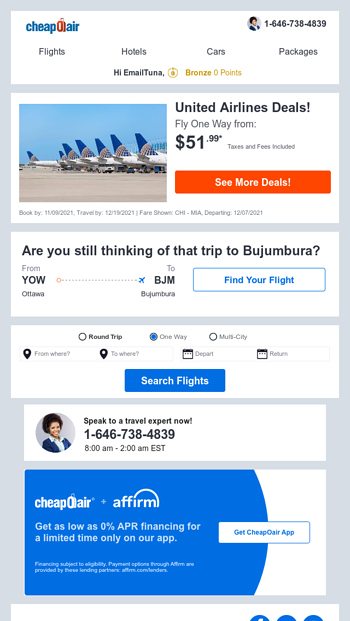The image depicts a mobile version of the Cheap Air website. At the top of the screen, a banner prominently displays the Cheap Air logo. Below the banner, users can navigate between options for flights, hotels, car rentals, and package deals. A contact number is provided at the top of the page, alongside a user icon with a 'Hi email' greeting, indicating a logged-in status with a Bronze zero points membership.

A featured advertisement highlights United Airline deals, offering one-way flights starting from $51.99. The ad showcases aircraft tails lined up on a tarmac against a clear blue sky, accompanied by a "See More Deals" button for further exploration.

Further down, another banner invites users to consider a trip from Ottawa to Bujumbura, featuring a "Find Your Flight" option. Just below, a search banner allows users to customize their travel plans by selecting round trip, one-way, or multi-city options. Interactive elements include dropdowns for departure and return locations, dates, and a map icon for additional help.

Near the bottom, a prompt encourages users to speak with a travel expert via a listed phone number, available from 8 AM to 2 AM Eastern Standard Time. The page concludes with an advertisement for a limited-time financing option exclusive to the Cheap Air app, encouraging users to take advantage of mobile-only offers.